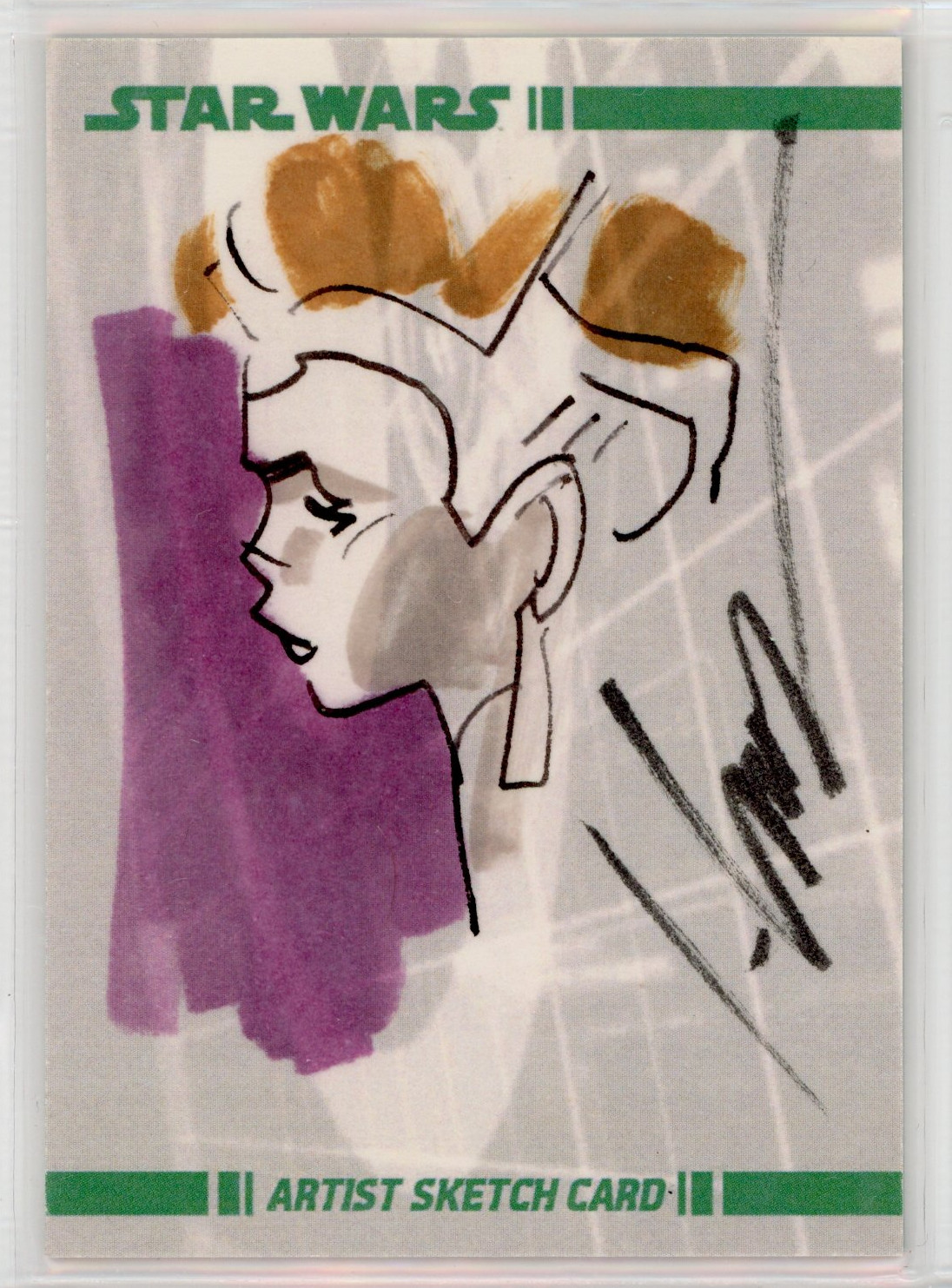This image appears to be an advertisement poster or a promotional artist sketch card with a predominantly grayish-white background. At the top, in green letters and underlined by a yellow line, it reads "Star Wars." The focal point is a black ink sketch of a female profile with very short dark brown hair, depicted simply and sparingly. Her head is adorned with strap-like headgear, and the background features a blob of purple on the left side and some black squiggly marks on the right, suggesting an abstract artistic style. The edges of the background have a rough, scratchy texture with white lines against the gray. At the bottom of the card, again in green letters, it says "Artist Sketch Card." Additionally, there is a vertically aligned artist's signature on the right side of the card.